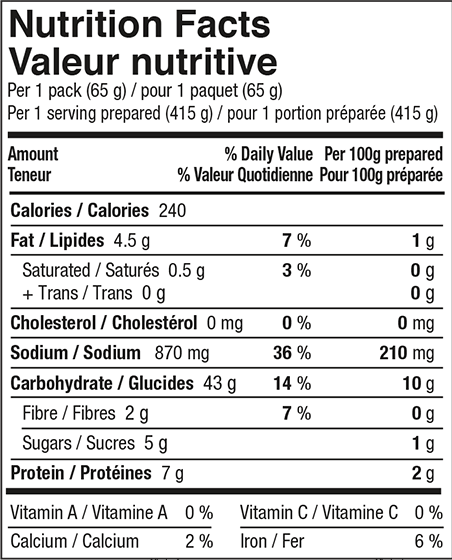This image is a close-up of a nutrition facts label that appears to be graphically made, possibly a screenshot. The label is presented in black text on a white background, with black horizontal bars separating different sections. At the top, it prominently displays "Nutrition Facts" in English and "Valeur Nutritive" in another language. The label provides detailed nutritional information for a single pack of a product, which has a serving size of 65 grams, and specifies the values per 100 grams prepared.

It states that each pack contains 240 calories. The breakdown includes 4.5 grams of fat (with 0 grams saturated and trans fat), 0 milligrams of cholesterol, 870 milligrams of sodium (36% Daily Value), and 43 grams of carbohydrates (including 2 grams of fiber and 5 grams of sugars). The pack also contains 7 grams of protein. For micronutrients, it shows 0% Vitamin A, 0% Vitamin C, 2% Calcium, and 6% Iron. The label does not specify the product type.